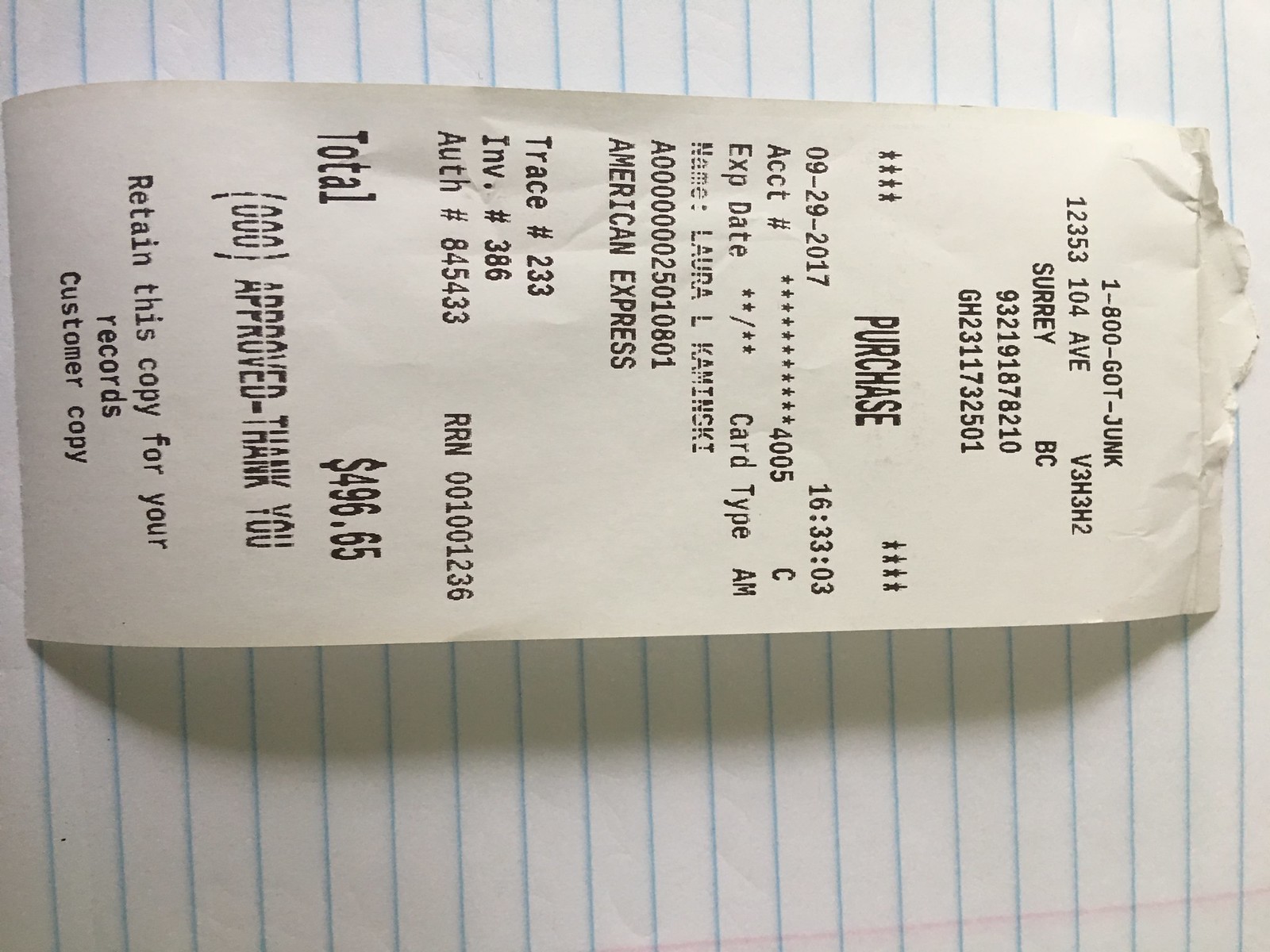The image depicts a photograph of a receipt laid sideways on a piece of college-ruled paper, with the bottom of the receipt facing the left side of the image and the top aligned with the right. The receipt is from the retailer 1-800-GOT-JUNK. The receipt lists extensive purchase details, including the date September 29th, 2017, and the military time 16:33:03. Payment was made using an American Express card by a person named Laura L. Kaminski. The total purchase amount was $496.65. The receipt also includes the store's address (12353 104 AV, Surrey, BC, V3H3H2) and various transactional codes such as a trace number (233), invoice number (386), and authorization number (845433). The words "APPROVED THANK YOU" and "RETAIN THIS COPY FOR YOUR RECORDS CUSTOMER COPY" appear at the bottom. The receipt is placed on a piece of loose-leaf paper with vertical blue lines.